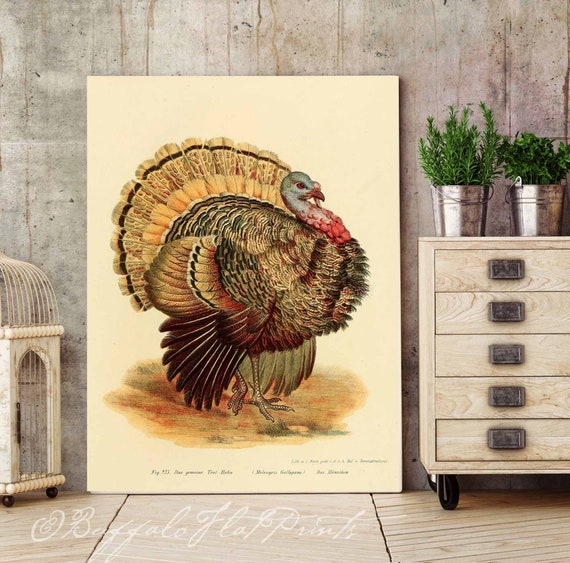This image features a detailed drawing or print of a wild turkey, prominently displayed on a large cream-colored poster. The poster, measuring approximately four to five feet in height, leans against a concrete wall. The setting includes a hardwood floor and, to the right of the poster, a chest of drawers. Two green plants, each growing in tin buckets, are placed atop the dresser. The wild turkey in the artwork is captured in a profile view, facing to the right, showcasing its detailed plumage and majestic stance. At the bottom of the poster, the artwork is credited to "Buffalo Flat Prints," though the exact text near the turkey is unclear.